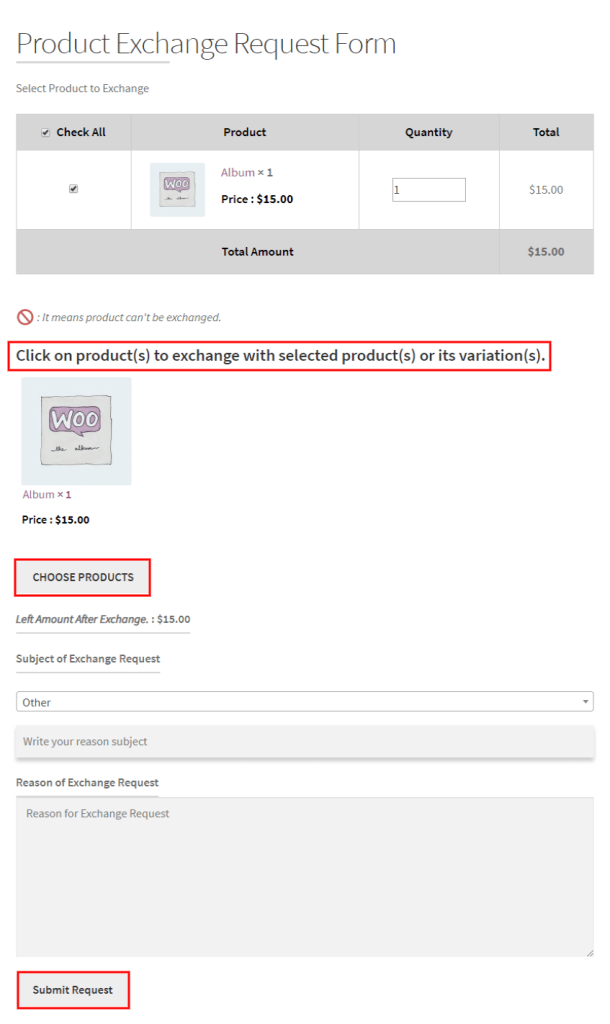This image depicts a screenshot of a product exchange request form. At the top, the heading "Product Exchange Request Form" is prominently displayed with an underline. Directly below, a prompt instructs users to "Select Product to Exchange." The checked product in this instance is "Album X1," listed at a price of $15 and a quantity of one, bringing the total to $15. 

A red circle with a line through it indicates that this product cannot be exchanged. Instructions suggest clicking on products to exchange them with selected products or their variations. Another entry for "Album X1" priced at $15 appears, and there is an option to "Choose Products." 

The form also shows the "Left Amount After Exchange" as $15, followed by fields labeled "Subject of Exchange Request" and "Reason for the Exchange." Users are directed to write their message subject and reason for the exchange in a text box provided for typing the exchange request's reason. 

At the bottom of the form, a "Submit Request" button is positioned for finalizing the request. Several key elements are highlighted with red boxes, notably the instructions "Click on Products to Exchange with Selected Products or Variations," the "Choose Products" option, and the "Submit Request" button. 

The form features a white background with black font for clear readability.